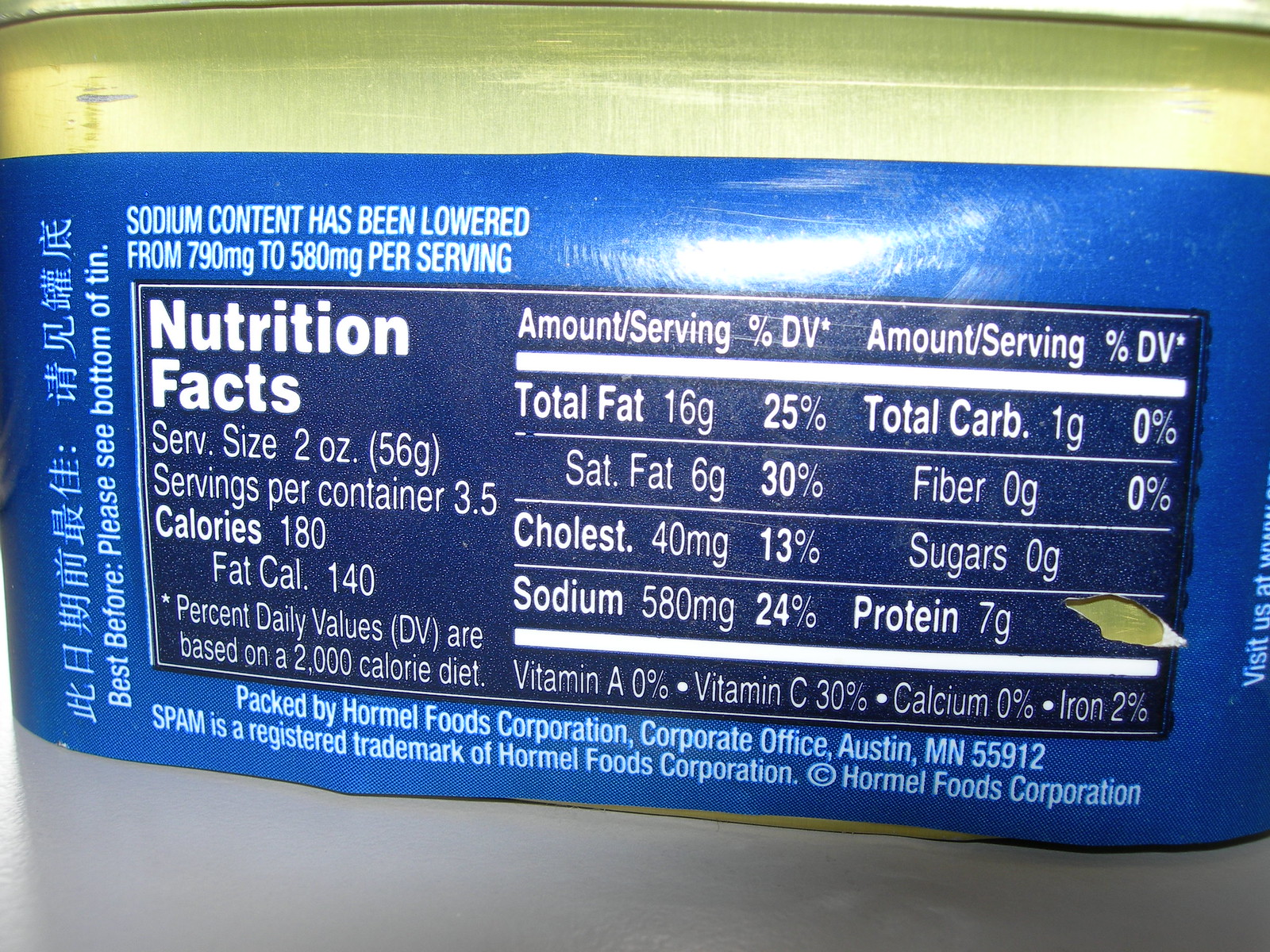The image features the back of a blue and gold can of SPAM, highlighting the nutritional label. The can is adorned with a blue band of paper and includes pertinent details such as the sodium content, which has been reduced from 790 milligrams to 580 milligrams per serving. The label specifies a serving size of two ounces, and the can contains three and a half servings. Additionally, the caloric information includes 180 calories per serving, with 140 of those being fat calories. Key nutritional values such as fat content, cholesterol, carbohydrates, fiber, sugar, and protein are clearly displayed. The packaging also notes that SPAM is a registered trademark of Hormel Foods Corporation, and there are Asian characters indicating "Best before, please see bottom of tin."